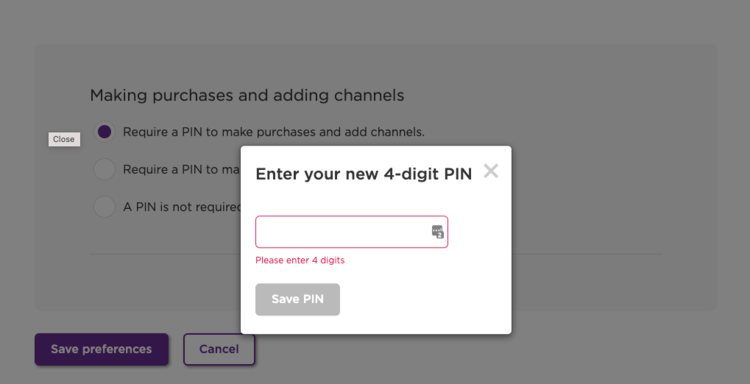The image depicts a Roku setup screen focused on configuring user preferences. The screen specifically displays options for managing purchases and adding channels. Users are presented with three choices: 1) "Require a PIN to make purchases and add channels," 2) an obscured option partially visible as "Require a PIN to...," and 3) another partially visible option where a PIN is not required.

The top choice, "Require a PIN to make purchases and add channels," is selected. Upon selecting this option, a white pop-up box emerges, prompting the user to "Enter your new 4-digit PIN" in a red-outlined field. The box includes a save button labeled "Save PIN" and an 'X' for closing the box. This step is mandatory to proceed with the setup, as closing the box without entering a PIN would prevent the user from saving their preferences. The alternative is to cancel the setup process altogether, implying the user might need to reconsider and finalize their decision at a later time.